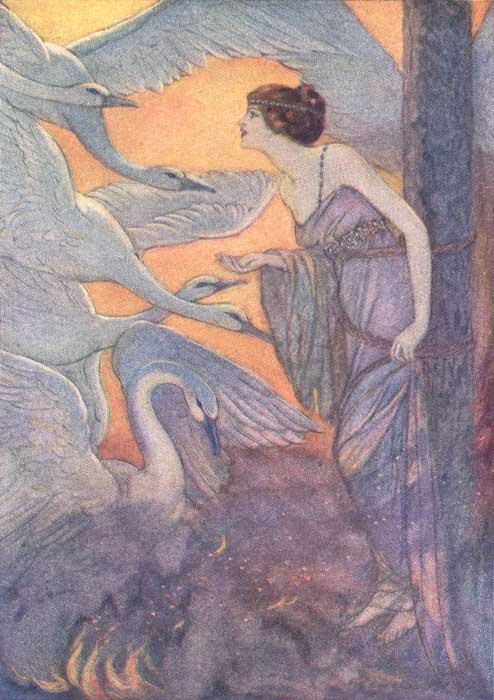The painting depicts a scene from Greek mythology, possibly Leda and the Swan, featuring a young white woman with slightly past-neck-length dark brown hair, adorned with a headband, and wearing red lipstick. She is dressed in a low-cut, thin-strapped purple dress, leaning forward against a pole with one hand on her hip and the other outstretched, as if offering something. Her figure dominates the right side of the image, barefoot and gracefully poised.

To the left of her, five swans with white to grayish feathers are flying toward her, their necks and wings outstretched in apparent friendliness. The background is a striking gradient of bright orange and yellow, reminiscent of a glowing sunset, contrasting with the predominantly purple hues that tint the rest of the artwork, including the soil-like foreground. There are also elements that could be interpreted as flames or a fire at the bottom of the image, adding to the mythical atmosphere of the scene.